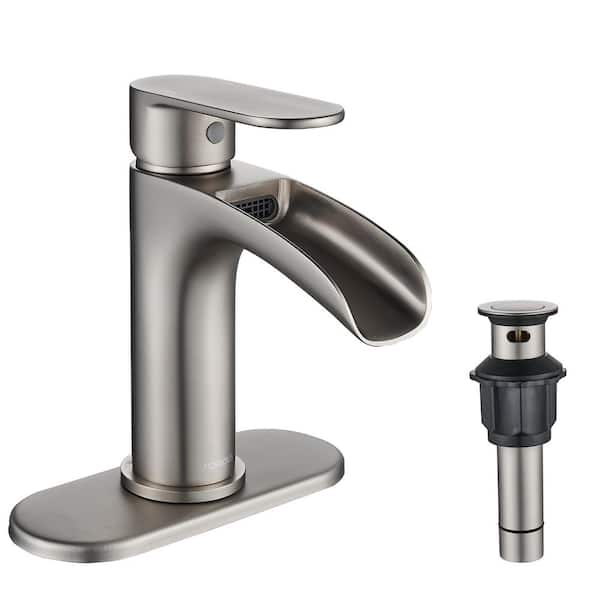The black-and-white photograph, set in a square format, prominently features a shiny, metallic kitchen faucet, positioned at an angle with its base towards the bottom left corner. The faucet exhibits a sleek, rectangular elliptical shape and a pewter-colored cylindrical stem that rises vertically. Atop the cylindrical stem is a flat, lever-style handle that users can lift up or down to control water flow. The spout, extending outward at a gentle angle, terminates in a finely curved lip, with a dark gray grate or mesh located near the outlet for water dispersion. To the right of the primary faucet, a secondary vertical element can be seen—a steel-like post with black caps at the top and middle, possibly serving as an extension or secondary filter. The background is stark white, emphasizing the faucet's detailed metallic texture and clean lines, presented in a style that blends representational realism with product photography aesthetics.